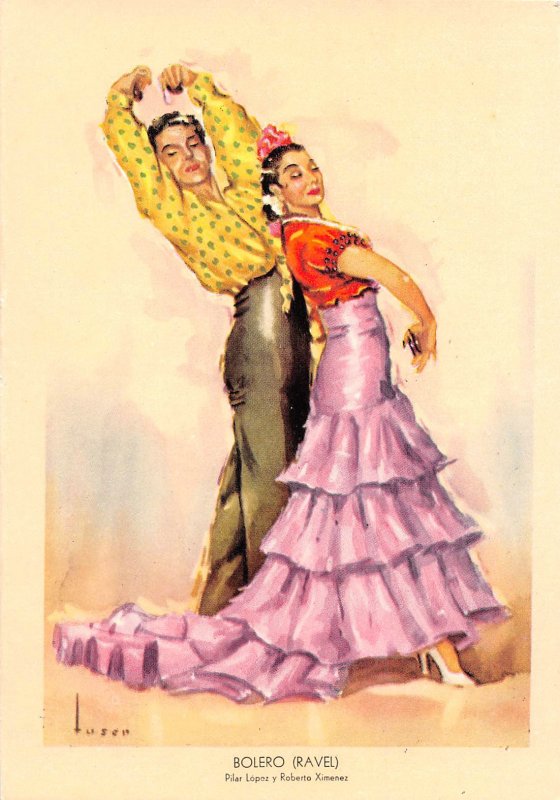A vintage hand-drawn illustration depicts two Spanish dancers named Pilar López and Roberto Jiménez, performing a traditional Bolero dance. The aged, sepia-toned paper and mottled background give it an antique, nostalgic quality, enhanced by an impressionist-style shadow cast around the dancers.

In the foreground, the female dancer, Pilar López, is adorned in a long, flowing, high-waisted pink ruffled skirt that puddles on the floor behind her. She wears a striking red top and white high heels that peek out from under her skirt. Her dark hair is styled with a red flower on top and a white flower in her ponytail. Red lipstick accentuates her face as she looks to the side, her right arm curved gracefully while holding castanets.

Standing slightly behind her, Roberto Jiménez, the male dancer, is dressed in shiny greenish-black high-waisted trousers and a yellow button-down shirt with green spots, which is open and tied at the waist. He leans backward, holding castanets above his head, his clean-shaven face and brunette hair completing his look.

At the bottom of the image, in black text, it reads: "Bolero Ravel, Pilar López y Roberto Jiménez," though the artist's signature on the left-hand side remains barely legible. The detailed and colorful depiction captures the movement and elegance of the dance, freezing a moment of cultural artistry in time.